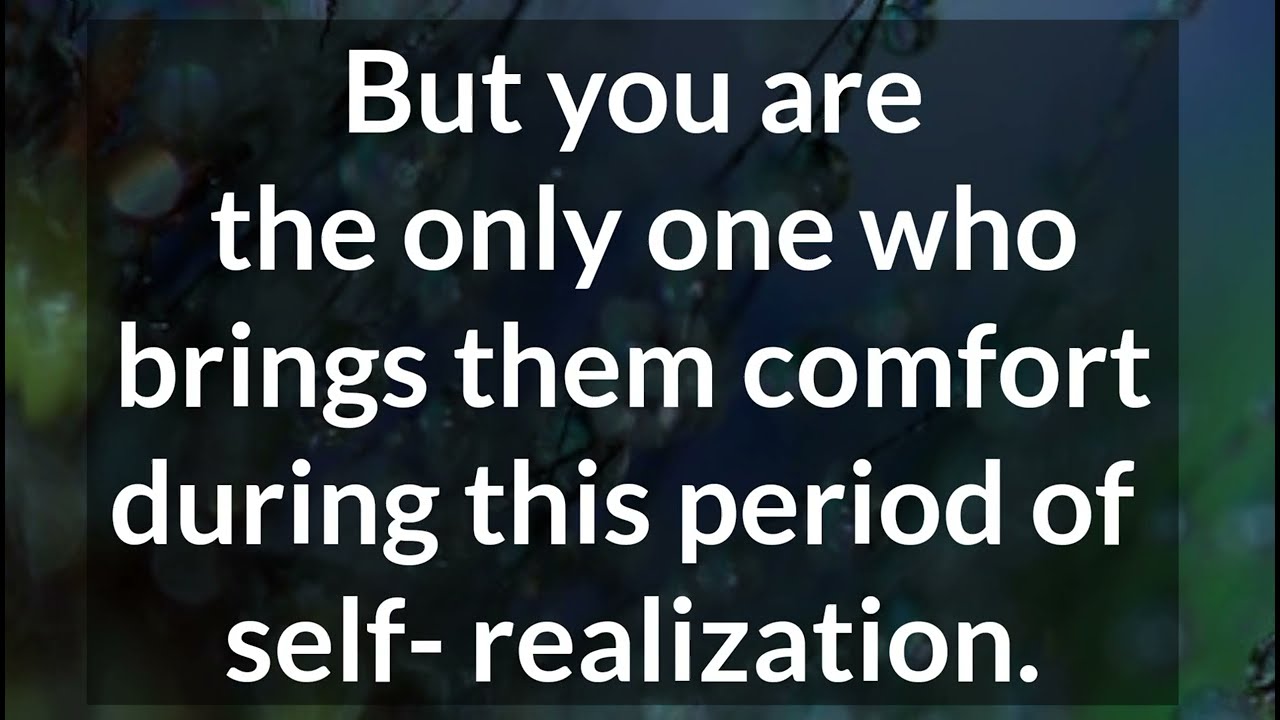The image is a motivational infographic, likely designed for a PowerPoint presentation or a video on spirituality or self-realization. At the center of the image, in a dark, semi-transparent rectangular text box, is a profound quote written in white text: "but you are the only one who brings them comfort during this period of self-realization." The text spans five lines and stands prominently over a blurred, serene background featuring green and blue hues, with suggestions of grass or tree branches. The background also contains shimmering lights or rainbow-like reflections, especially visible on the far left, adding an ethereal quality to the overall composition. The entire image is rectangular, with its edges appearing slightly brighter than the area behind the text box.